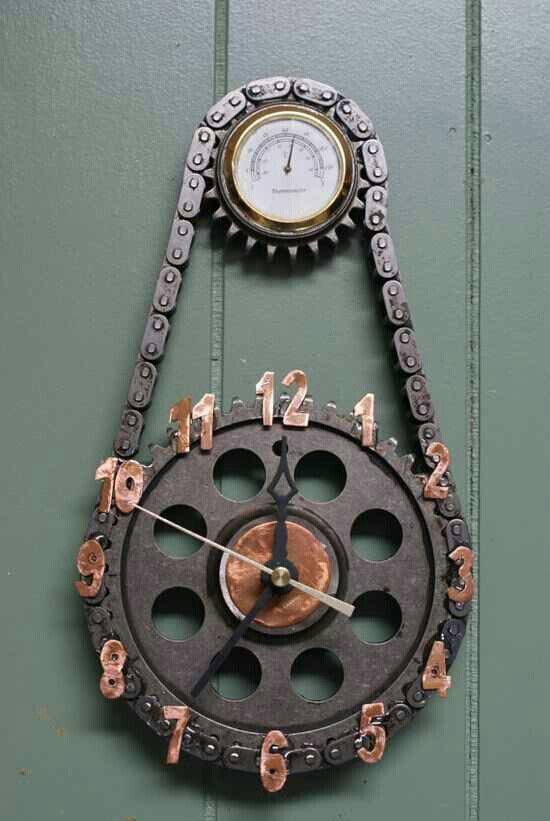The image depicts a partially green and gray wall, adorned with various lines and textures. Centered at the top is a round meter which features a series of numbers arranged in a circular pattern. Surrounding this meter is a chain that loops around it, bordered by gear-shaped markings along its exterior.

The chain, meticulously illustrated with elliptical dots, connects to a significant gear at the bottom of the composition. The meter's face is detailed with small holes and appears weathered, with visible signs of rust. The hour hand is fixed at the 12 o'clock position, while what seems to be the second hand points to 10, distinguished by its white coloration. The minute hand rests at 7 o'clock. 

The entire wheel, painted in black, is numbered from 1 through 12. Each numeral exhibits a patina of rust, adding to the overall vintage and industrial aesthetic of the piece.